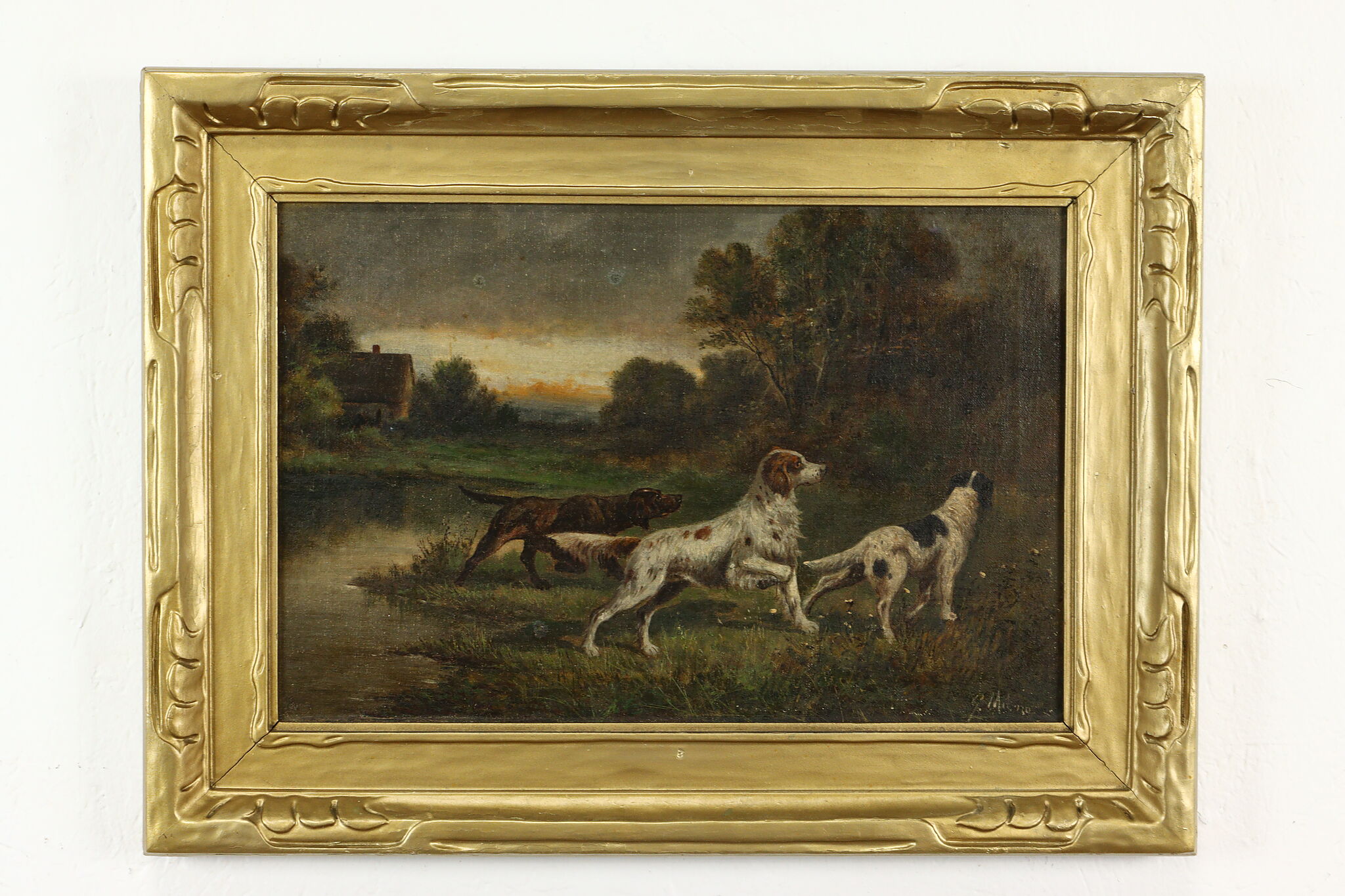The image is a photograph of a painting, prominently displayed on a white wall with a thick, gold-colored frame. The painting features a realistic, classic scene likely created with oils. In the foreground, three dogs—two white with different color patches and one brown—are intently looking to the right, appearing to be hunting or focusing on something in the distance. They are situated on a grassy area by a lake, with a rustic cabin visible in the background. Surrounding them are trees and pockets of woods under an overcast, possibly sunset sky that hints at an impending storm. The natural setting, including the water and trees, adds depth to the painting, creating a nostalgic portrayal of dogs in the wilderness.